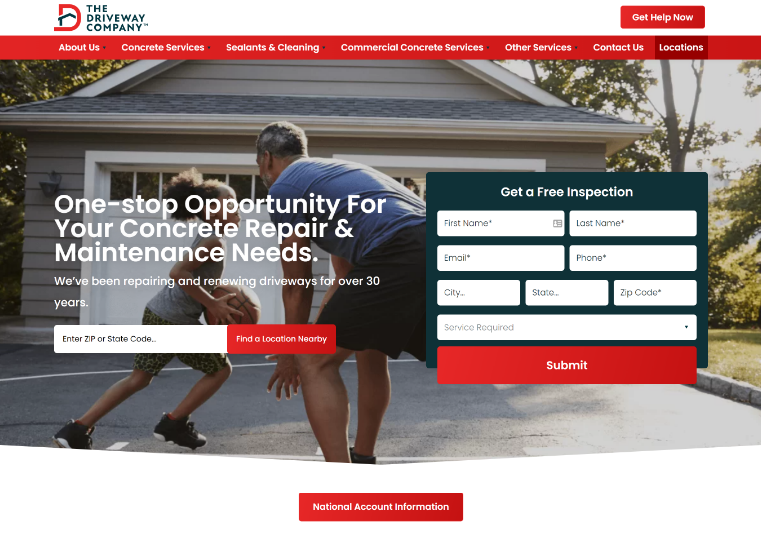The website for the driveway company features a clean, predominantly white design. The logo is distinctive, with a 'D' that wraps around a stylized roof, presumably symbolizing a garage rather than a driveway. To the right of the logo, a prominent call-to-action button reads "Get Help Now," guiding users who are seeking driveway services.

At the top of the page, a red navigation bar lists several clickable links: About Us, Concrete Services, Sealants and Cleaning, Commercial Concrete Services, Offer Services, Contact Us, and Locations. Currently, the Locations section appears to be selected.

A large image captures attention below the navigation bar. It depicts a standalone two-car garage with a driveway, which intriguingly has basketball court lines painted on it. In the foreground, an older man, possibly a grandfather, is playfully guarding a young girl who holds a basketball with both hands, about to take a step.

Text overlaid on the image highlights the company’s expertise: "One-stop opportunity for your concrete repair and maintenance needs." In white letters, it announces, "We’ve been repairing and renewing driveways for over 30 years." There is a form prompting users to enter their zip code or state code to find a nearby location. Additionally, a section allows for a free inspection request by submitting personal details including first name, last name, email, phone, city, state, zip code, and specific service requirements. 

This comprehensive and user-friendly website offers valuable information and services, ensuring visitors learn all they need to know about the driveway company.